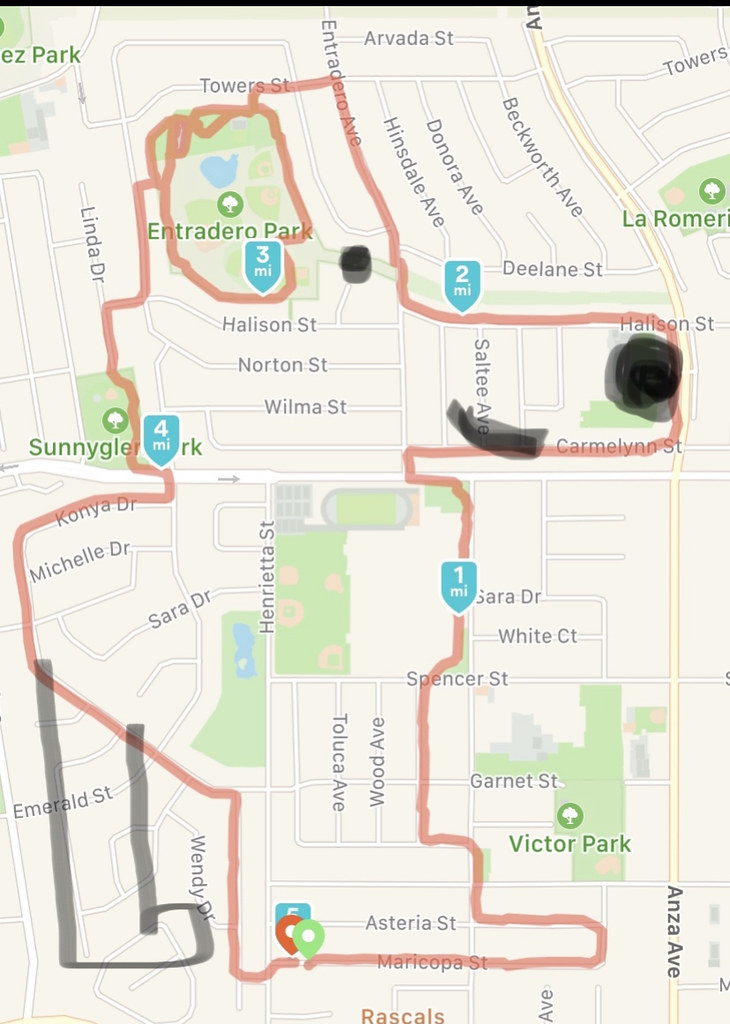This detailed map illustration highlights a specific route through a network of parks and streets. At the upper left corner, Intradero Park is prominently outlined in red, featuring a marker indicating a distance of three miles. This park connects to other parks via red lines. To the left, these lines lead to Sunny Glare Park, partially obscured by a blue and white ticker indicating 4 miles and marked RK. 

Additionally, another red line extends downward from Intradero Park, branching off near the west edge of the map. Here, a black line diverges near the intersections of Michelle Drive, Sarah Drive, and Emerald Street. At the bottom of the map, two markers, one neon green and another red-green, are positioned where the line ends before resuming its northward trajectory.

In the lower right area of the map, Victor Park is noted near Garner Street, accompanied by a one-mile marker heading north. A black blob is drawn near Hallison Street in the upper right portion of the map. Toward the right edge, part of La Ramerie Park is visible, and running down the entire right side is Onza Avenue, highlighted in yellow.